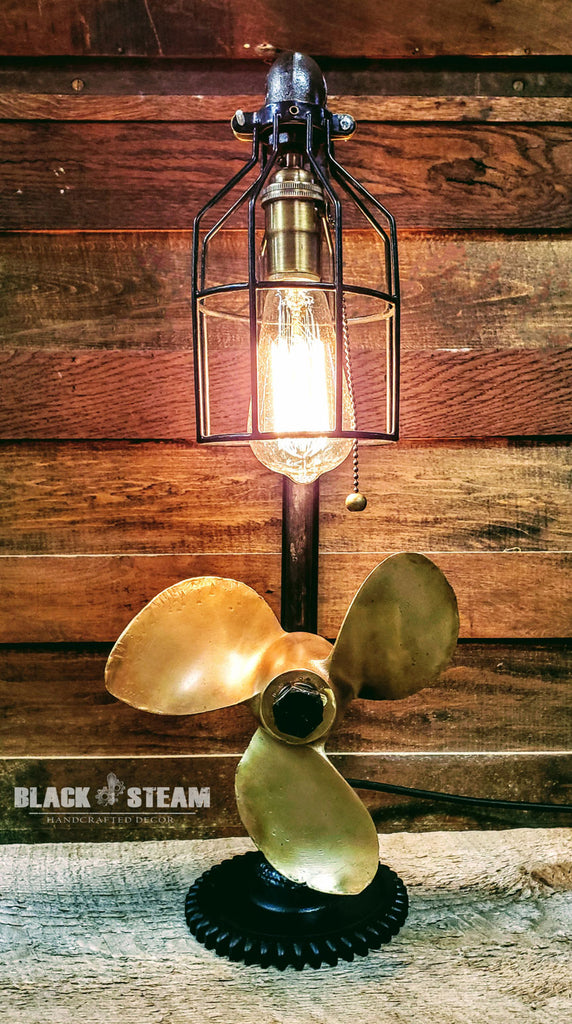The image features a vintage-styled lamp with an integrated fan at the bottom, characterized by its open wire design and antique ambiance. The lamp, situated on a lighter colored wooden table, stands against a reddish-brown plank wall in the background. The fan attached to the lamp features three gold metallic blades and is positioned just above the lamp's black stand. The lamp boasts a distinctive old-fashioned, elongated Edison bulb operated by a pull chain. In the lower right corner of the image, there is some barely readable text that includes the words "Black Steam" with a small, indistinct icon between them. The lamp and fan ensemble exudes a handcrafted, nostalgic décor aesthetic.